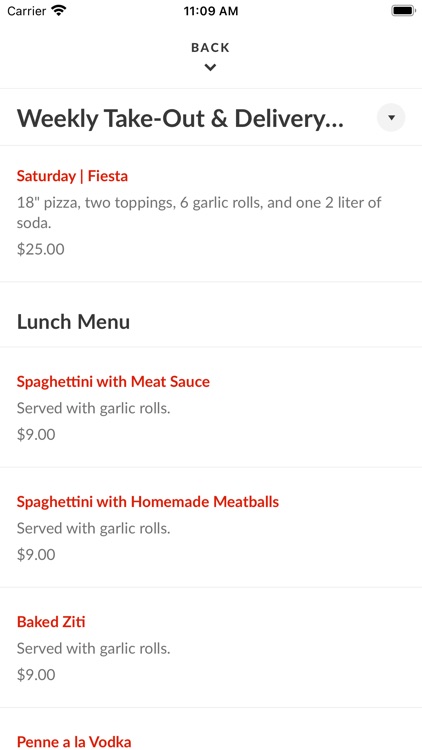A detailed caption for the provided image description:

The screenshot captures a mobile device display showcasing a restaurant app's takeout and delivery menu. The device indicates full Wi-Fi strength and the time is 11:09 AM, with the battery nearly fully charged. At the top of the screen, there's a headline in bold text reading "Weekly Takeout and Delivery". Below the headline, red text highlights a promotional deal saying "Saturday Fiesta". Underneath, gray text details the offer: "18 inch pizza, two toppings, six garlic rolls, and one two-liter soda for $25".

Subsequent information includes a section labeled "Lunch Menus" in black text. The first item listed in red is "Spaghettini with Meat Sauce", with gray subtext noting that it is "served with garlic rolls". Following this, another item described in red text reads "Spaghettini with Homemade Meatballs served with garlic rolls $9", and then "Baked Ziti served with garlic rolls $9". The final menu item partially visible at the bottom, written in red text, is "Penne a la Vodka", but the accompanying gray subtext is cut off. At the top center of the screen, a back button is also visible.